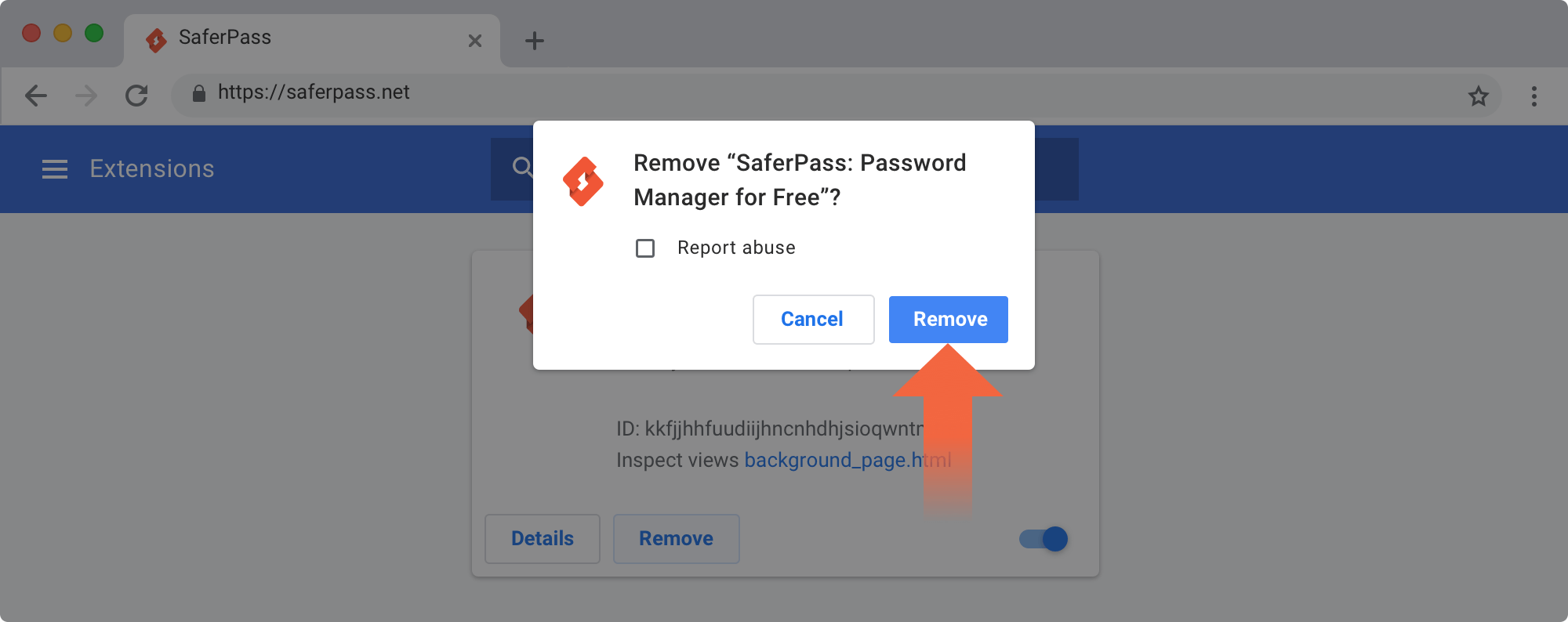This image, sourced from the website saferpaths.net, prominently features a control panel-like layout. On the left side, there are three circular icons: a red circle, a yellow circle, and a green circle, likely representing some form of status indicators. Adjacent to these circles is a series of buttons, including a gray left arrow button, a right arrow button, and a refresh button. Further to the right, we see a star icon and an icon consisting of three vertical dots, indicative of more options.

Superimposed on the screen is a notification pop-up asking, "Remove SaferPaths Password Manager for free?" The pop-up includes three clickable buttons: a report abuse button, a cancel button, and a prominent blue-and-white remove button. A large red arrow is directing attention towards the remove button. Below this pop-up, there is a display of what seems to be a long ID number, formatted as KKFJJHHFUUD. The overall layout suggests a user interface related to password management or digital security.